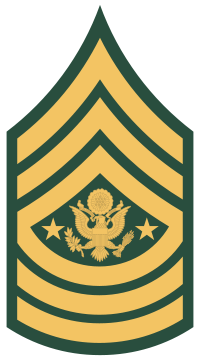The image features a computer-generated depiction of a U.S. Army Command Sergeant Major insignia, presented on a white background. This insignia, likely used to denote rank, has a distinctive shape with a triangular top that transitions into a tube-like structure rounded at the bottom. The patch is outlined in green and contains a series of gold-colored elements. At its center, an American Eagle is prominently displayed, clutching an olive branch and arrows in its talons. The eagle is flanked by two golden stars and topped with a golden circle. Above and below the eagle are sets of stripes: three at the top and two at the bottom. The entire design showcases intricate decorative trim, emphasizing the prestigious military rank it represents.